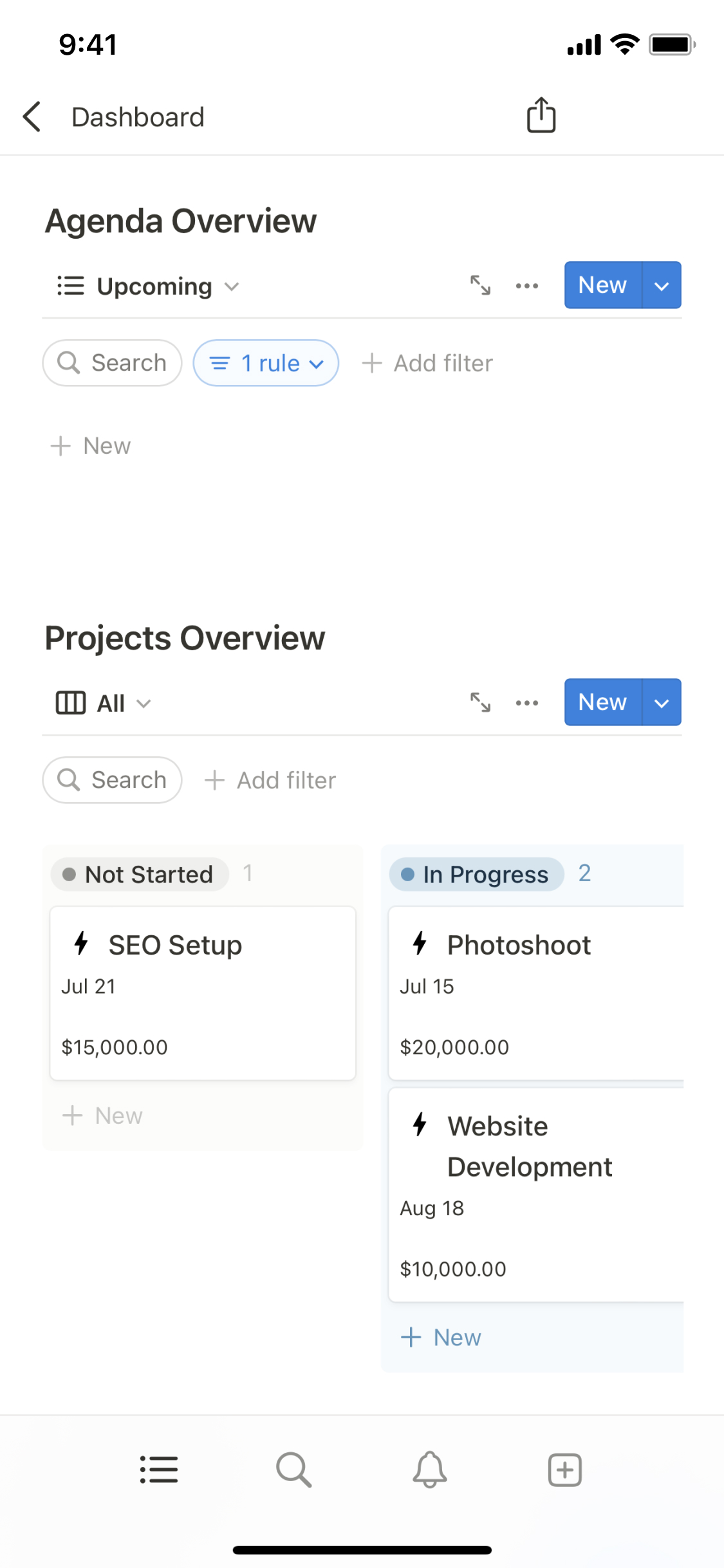The screenshot of a cell phone display showcases various interface elements and status indicators. At the top of the screen, the time is displayed as 9:41, accompanied by four bars of cellular signal strength, a full Wi-Fi signal, and a fully charged battery icon. 

Directly below the status bar, there is a back arrow icon pointing to the left beside the word "Dashboard" in gray text. The main content area of the screenshot begins with a heading titled "Agenda Overview." Beneath this heading, there is a section labeled "Upcoming," with a blue square button on the right that says "New."

Further down, there is a set of interactive options including a search bar, a "one rule" filter, and an "Add Filter" button. The subsequent section is labeled "Projects Overview." Within this section, there is a selection field marked as "All," and to its right, another blue box labeled "New."

The bottom part of the screen is divided into four square sections, each representing different project statuses. The first square is labeled "Not Started" and displays the project "SEO Setup," scheduled for July 24th with a budget of $15,000. To the right of this, the "In Progress" section showcases two projects: a "Photo Shoot" with a budget of $20,000 and "Website Development" with a budget of $10,000.